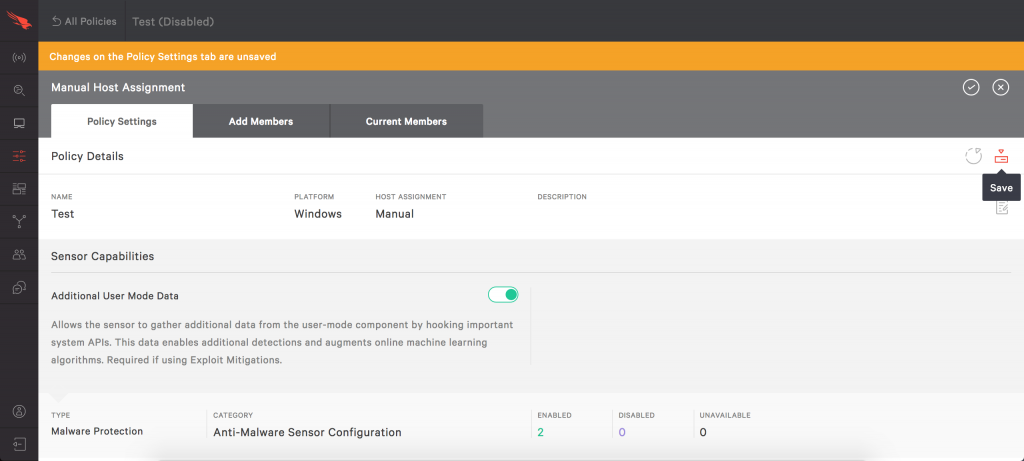The image is a screenshot of a user interface featuring a sidebar and various widgets labeled with small, mostly indistinguishable text.

On the left-hand side, there is a prominent black vertical bar. At the top left corner of the bar, there is an indiscernible red icon followed by two small gray elements whose details are not clear. Below these, there are additional gray items and a lighter gray item, all too small to make out. Continuing downward, there are red lines, several more gray elements, and then two final gray elements at the bottom.

At the top of the image, there is a dark gray rectangle with an unidentified gray symbol and unreadable gray text. Below this are an orange rectangle with white text and a gray rectangle with white text. 

On the right side, there are two circles; one contains a check mark and the other an X. Adjacent to these circles, there are three tabs: a white tab labeled "Policy Settings," a gray tab labeled "Add Members," and another gray tab labeled "Current Members." Below these tabs, there is a section titled "Policy Details" with additional small, unclear text on a white background.

To the far right, there is a red symbol and a black rectangle with a small triangle on top labeled "Save." Below this, a gray rectangle contains unreadable text, followed by more indiscernible text in smaller gray rectangles beneath it.

In the center of the image, there is a green-outlined shape with a green dot on its right side and more unreadable text. Additionally, there is a light gray rectangle with small, indistinguishable text, and at the bottom, there are three numbers; one in green and the other two in black.